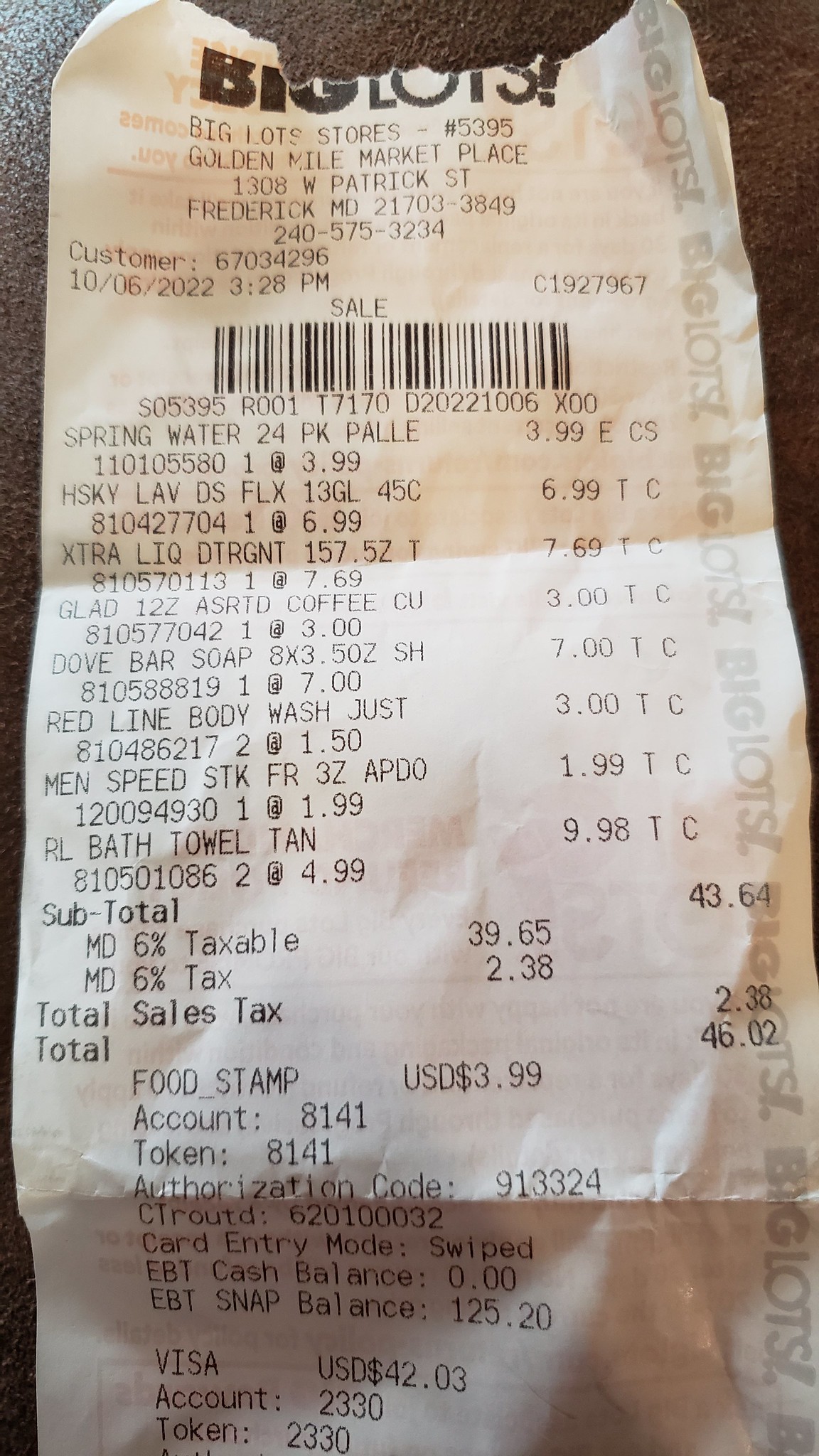This color photograph depicts a crumpled receipt with black text on a white background, lying on a greyish-brown surface. Prominently featured at the top is the store name "Big Lots" in bold print. Below that are smaller, less legible details including various items listed with their corresponding prices. Clearly visible is an entry for "Red Line Body Wash," priced at $3.00 for two units at $1.50 each, and "Men's Speed Stick," available for $1.99. The subtotal of the purchases is $39.65. Sales tax is calculated at 6%, amounting to $2.38. A note indicates that food stamps were used for a $3.99 payment. The bottom portion of the receipt is more difficult to decipher due to its crumpled state, while a fold at the top further complicates readability. A grey watermark runs vertically along the right-hand side, adding to the visual clutter.